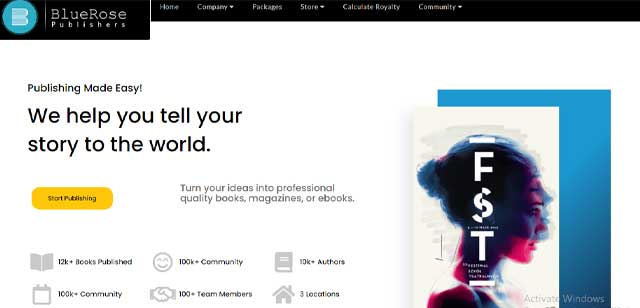The header of the website prominently displays "Blue Rose Publishers" in large, white text, indicative of a digital book publishing company. Accompanying the text is an artistic bee logo encased in a blue circle. Positioned on the right side in smaller, white text on a black background are navigational links: "Home," "Company," "Packages," "Store," "Calculate Royalty," and "Community."

Below the header, a white background features the phrase "Publishing made easy!" in a bold 8-10 point font. Below this, in much larger text, appears the empowering statement, "We help you tell your story to the world." Adjacent to a noticeable yellow "Start Publishing" button is the encouraging text: "Turn your ideas into professional quality books, magazines, or e-books."

Further down, the site showcases six distinct images underlining its achievements and offerings. They proudly display milestones such as "12,000+ books published," indicated by an open book emoji, a smiley face representing a "100k community," and "10,000+ authors." They also highlight a team of "100+ members" across three locations.

On the right side of the page, there is a featured book with a distorted side-view portrait of a woman. Above her image, the text "FST" is positioned alongside a striking blue border.